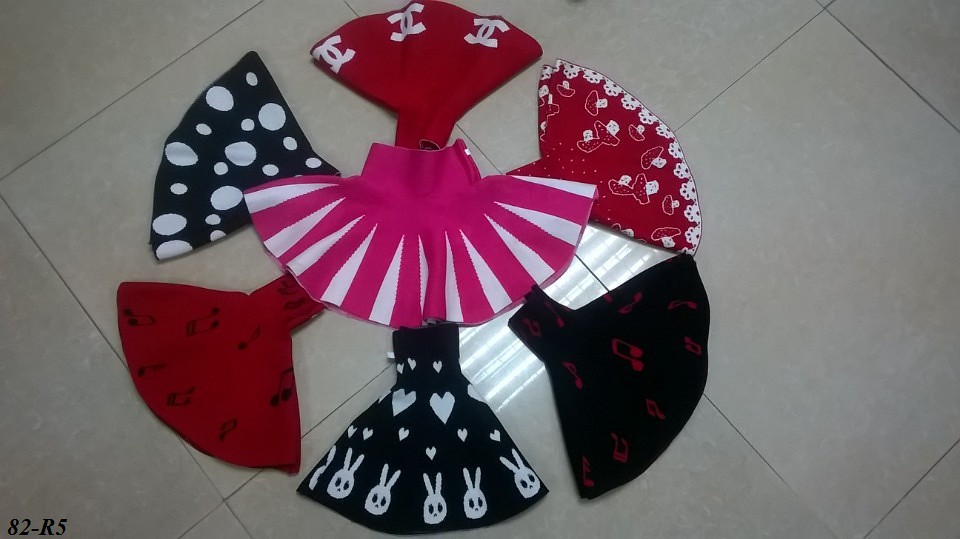In this image, seven vintage-style skirts are arranged on a white-tiled floor, forming a circular pattern with their waistbands inward and hemlines outward. The skirts include a variety of designs: starting from the bottom and moving clockwise, one black skirt features white hearts and bunny rabbit faces; a red skirt displays musical symbols; another black skirt is adorned with white circles; at the top, a red skirt showcases the Chanel logo; following it is a red skirt with white flowery symbols and mushrooms; and finally, another black skirt has red musical symbols. In the center of the circle, there is a dark pink skirt with white lines, resembling a cheerleading skirt. The floor is illuminated by the reflective glare of ceiling lights, and in the bottom left corner, there is a marking "82-R5" in black, contributing to the vintage ambiance.